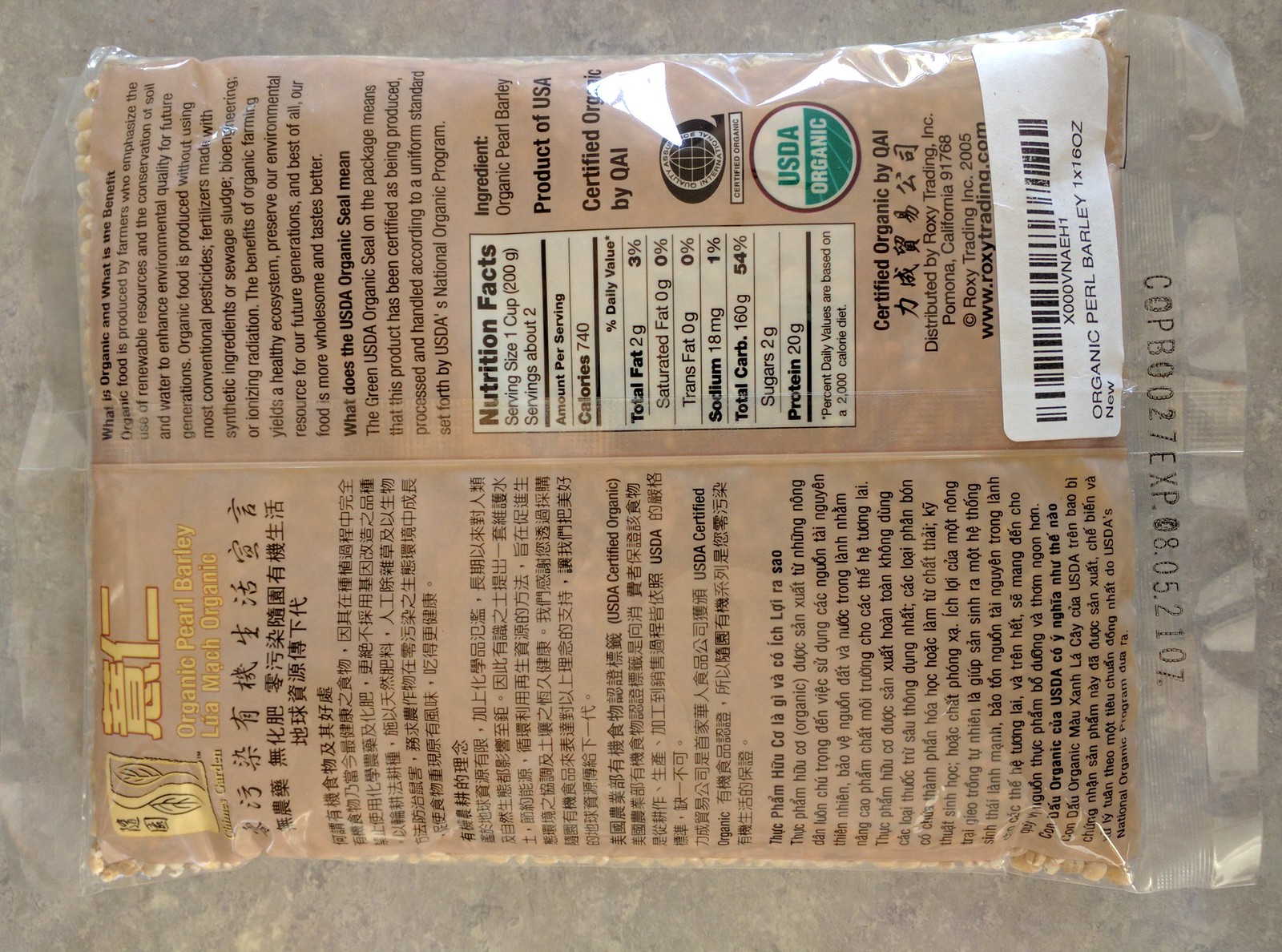This photograph showcases the back of a bag of Organic Pearl Barley placed sideways on a light gray granite countertop. The product originates from China, as indicated by the packaging. The bag prominently features a yellow logo adorned with Chinese script and two leaves, along with the English text "Organic Pearl Barley." Additional Chinese script surrounds the logo, accompanied by translated text in another language. A small Nutrition Facts label confirms that the product is organic and produced in the USA. At the bottom of the bag, a barcode sticker with the product name "Organic Pearl Barley" and a series of numbers is also visible. The image focuses solely on the bag against the granite surface, with no other objects in view.